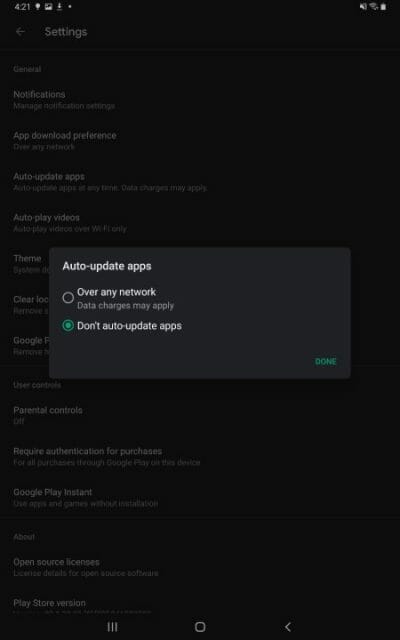Here’s a cleaned-up and detailed caption for the image:

---

The image appears to be a blurry screenshot from a mobile device, possibly a tablet or phone, displaying a settings screen. The background is predominantly black with greyed-out text. A central window, slightly lighter in shade, is the focus of the image. 

At the top left of this window, the title "Auto-update apps" is visible. Below this title, two options are presented: "Over any network," which is not selected, and "Don’t auto-update apps," which is marked by a green circle indicating it is selected.

The overall image quality is poor, making finer details hard to discern even at 200% zoom. Some elements can still be identified: "Settings" is greyed out and located in the background at the top left corner. The time displayed on the device is 4:21. There are some indistinct icons, likely phone-related, at the top of the screen.

Additional settings options are somewhat readable, including "General settings," "Notifications," "App download preferences," "Auto-Update apps," "Autoplay videos," and possibly "Teams" along with other unidentifiable items. The phrase "Clear something" and "Google" are partially visible, and "done" appears in green at the bottom right edge of the central window.

Further down, terms like "Require authentication for purchases," "Google Play," and something that begins with "Variant," followed by an illegible string, are present. The bottom of the screen holds three navigation buttons: a vertical three-line button (likely for menu access) on the left, a central round home button, and a back button on the right.

Overall, the image remains very dark and blurry, hindering detailed readability.

---